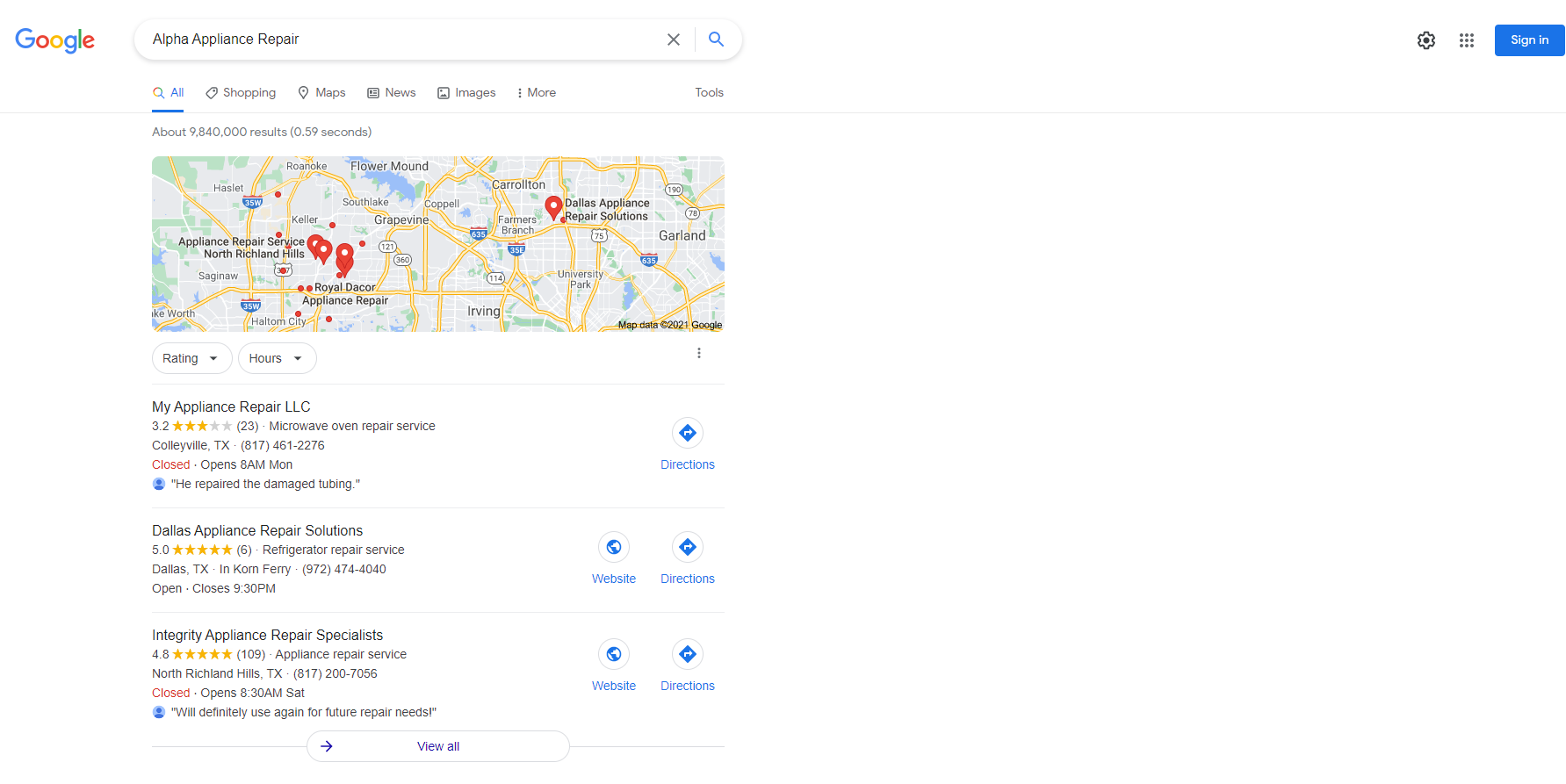A detailed screenshot of a Google search page featuring a search for "Alpha Appliance Repair." At the top-left corner, the iconic Google logo is displayed in colorful, rainbow letters. Adjacent to the logo is the search bar with the queried text "Alpha Appliance Repair." 

Below the search bar, several navigation tabs are visible, starting with "All," which is highlighted in blue to indicate the current selection. The other tabs, written in black, include "Shopping," "Maps," "News," "Images," "More," and "Tools," stretching from left to right. A subtle light-gray line separates these tabs from the search results. Beneath this line, it is noted that there are about 9,840,000 results displayed in 0.59 seconds.

The first prominent feature on the results page is a rectangular map with various pinpoints indicating appliance repair services. On the left side of the map, notable pinpoints include "Appliance Repair Service, North Richland Hills," and "Royal Decor Appliance Repair." On the right side, there is a pinpoint for "Dallas Appliance Repair Solution."

Directly below the map, two buttons with drop-down menus allow users to filter results by "Ratings" and "Hours." Finally, three appliance repair businesses are listed beneath these buttons: "MyApplianceRepair," "Dallas Appliance Repair Solution," and "Integrity Appliance Repair Specialist."